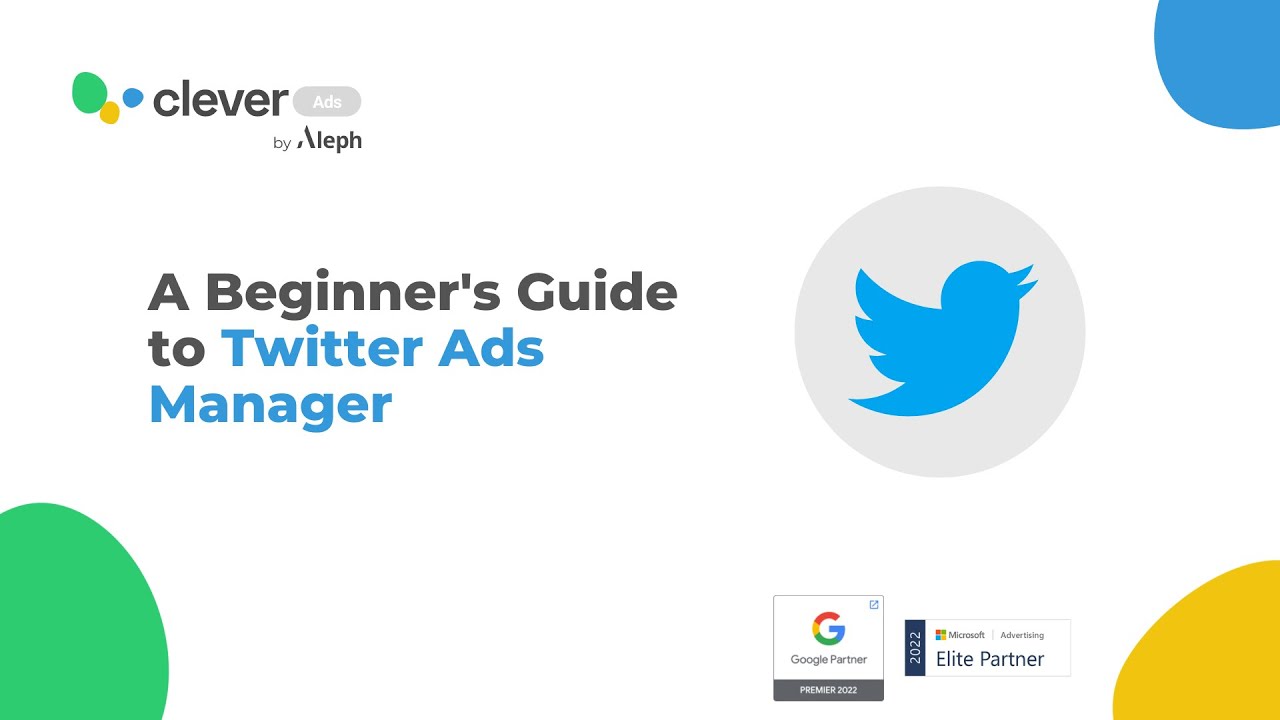This image is a cropped screenshot of an informational graphic or advertisement by Clever Ads, a brand by Aleph. The top-left corner features colorful, overlapping bubbles in green, blue, and yellow, with "Clever" prominently written in large black font to their right. Adjacent to "Clever," a grey bubble displays the word "Ads" in small white font. Below this, "by Aleph" is printed in large black letters. The ad's background is a clean white.

At the top right corner, there's a blue bubble, while a green bubble occupies the bottom left corner and a yellow bubble is positioned in the bottom right corner. Near the center right of the page, a substantive grey bubble prominently features the blue bird logo of Twitter. To its left, the phrase "A Beginner's Guide to Twitter Ads Manager" is displayed, with "A Beginner’s Guide To" in large black letters and "Twitter Ads Manager" in large blue letters.

In the bottom right corner of the image, there are two icons: one representing Google Partner and the other signifying Microsoft Elite Partner.